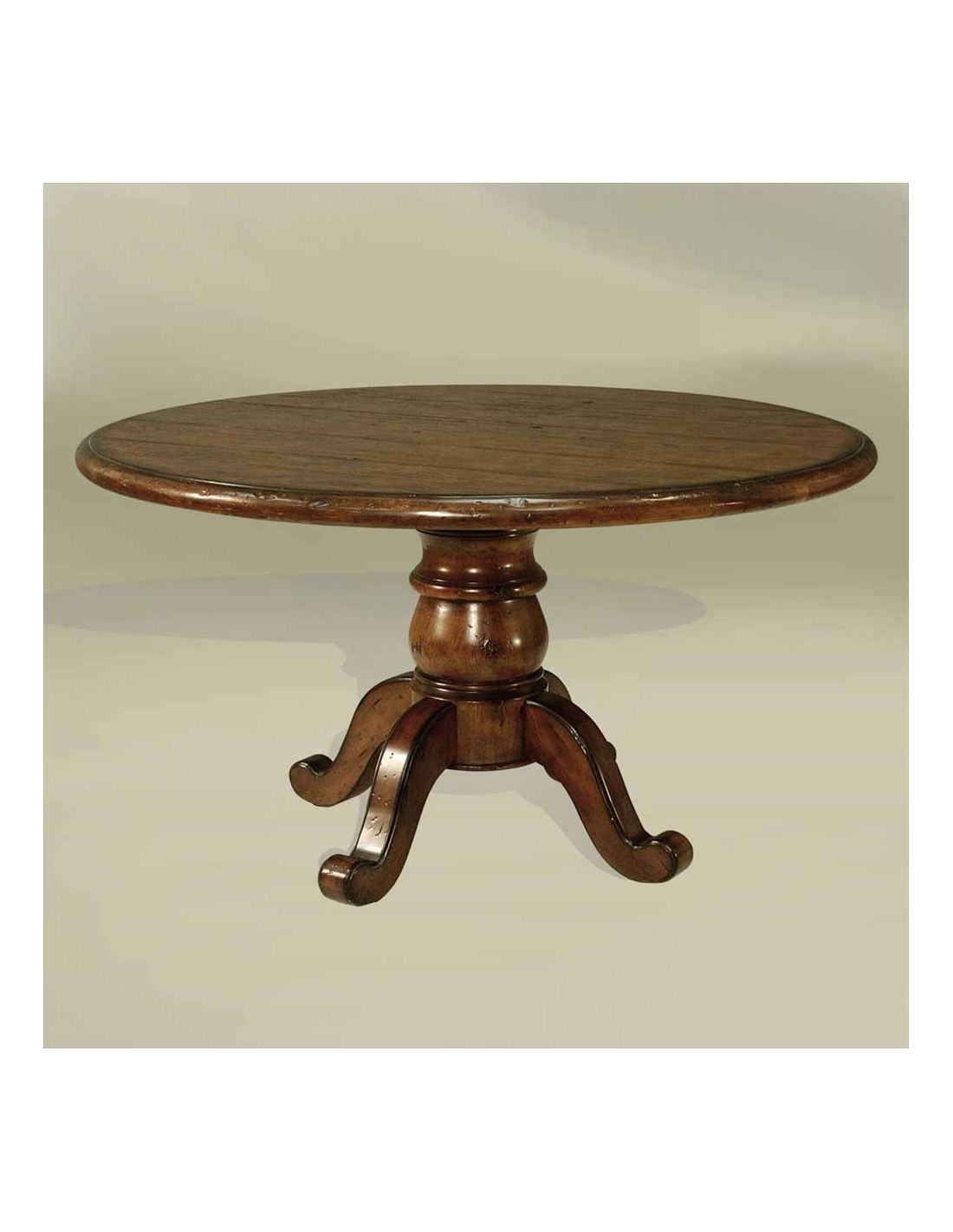This photograph captures a close-up of a cylindrical wooden table standing on a white surface with a matching white background. The table's top is made of simply finished wood, showcasing a clear contrast to the edges and base, which are treated with a shiny, more vibrant brown finish. The edges of the tabletop are rounded and smooth, adding a subtle elegance to the design. The table is supported by a distinctive base that features curved legs forming a half-S shape, connecting to a circular pedestal that tapers up like a piece of pottery. This pedestal consists of three segmented parts: the first is circular with all the legs attached, the second tapers upwards into a bowl-like shape, and the third tapers down to fit seamlessly with the table surface. The shadow of the table is cast to the left, adding depth to the minimalist white setting.